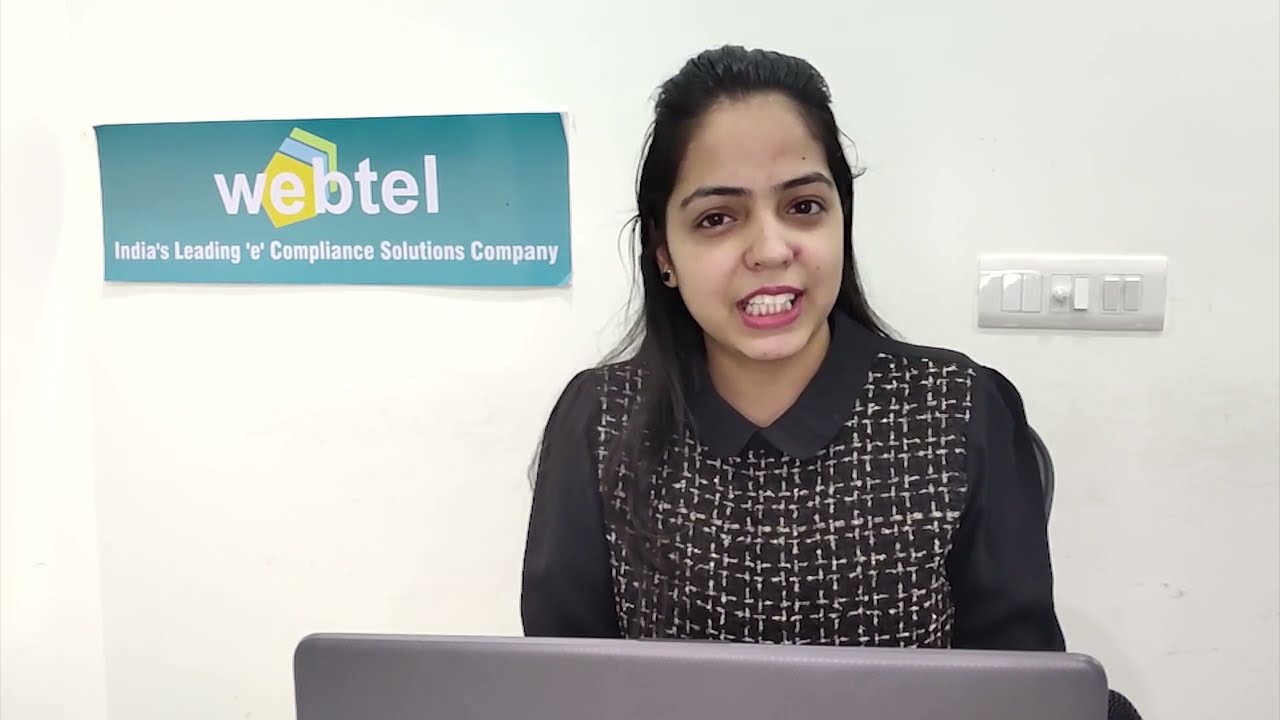This image captures a South Asian woman, likely in the middle of a conversation or presentation, as her mouth is open. She sits behind a partially visible gray laptop. The woman is dressed in a black long-sleeve shirt with a unique pattern of tan sketches resembling disjointed stripes, and she has a black collar. Her dark, straight hair is partially pulled back, and she wears black stud earrings. Her fair complexion is complemented by bright red lipstick and dark brown eyes. To her right is a white wall featuring a white panel with multiple light switches, and to her left is a blue advertisement banner. The banner reads "WEBTEL" at the top in white text, followed by "India's leading e-compliance solutions company." The logo on the banner comprises pentagons in green, blue, and yellow, positioned behind the letter 'E' in "WEBTEL."